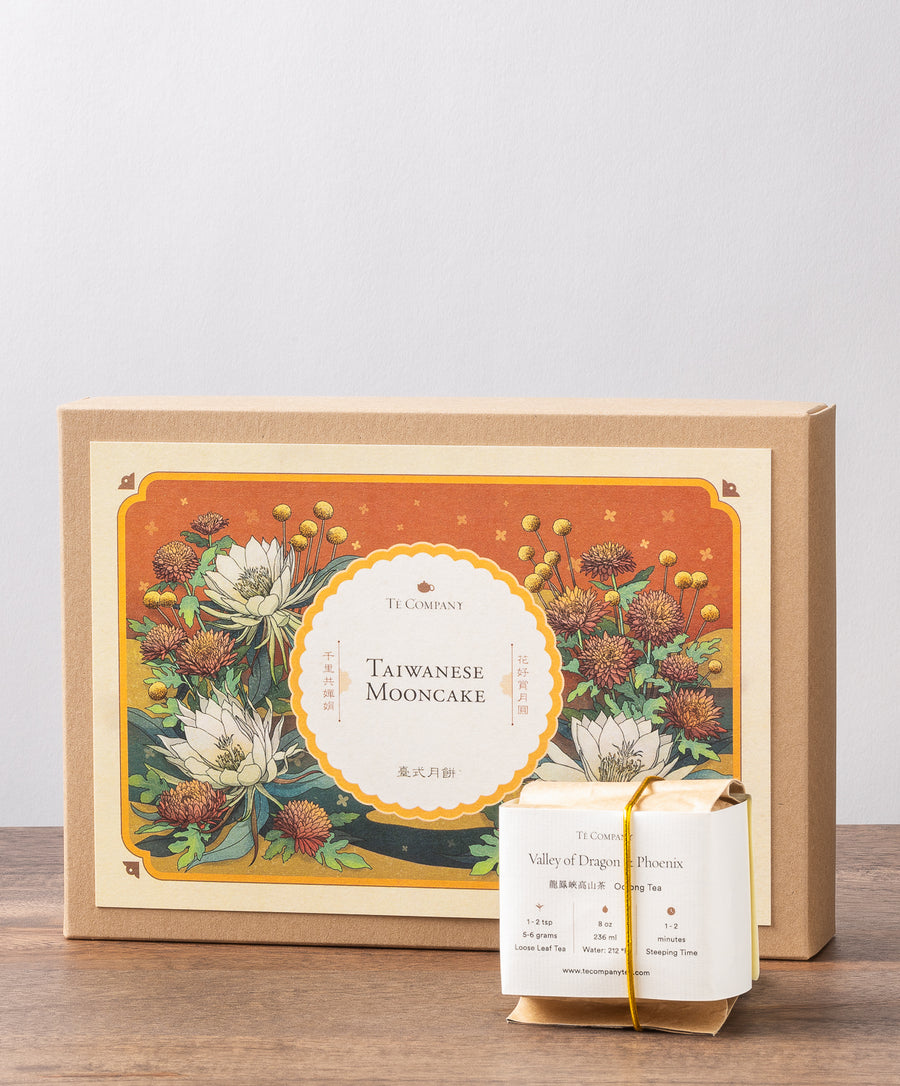The image showcases a display set on a light-colored wooden table against a white wall. Central to the scene is a brown box adorned with intricate flower illustrations in a palette of whites, yellows, muted tans, and browns. The background design of the box grades from orange to yellow, eventually blending into a grayish-blue near the bottom. Prominently featured on the box is a scalloped circle with a yellow edge and white center inscribed with "Taiwanese Mooncake" surrounded by Asian characters. This box, standing upright, displays the logo of the Tea Company (TE Company), including a teapot graphic.

Next to the main box, slightly in front and to the right, rests a smaller package wrapped in brown paper and tied with a golden ribbon. This package, labeled "Valley of Dragon and Phoenix," provides detailed instructions for tea preparation, including the required tea amount, water quantity, and steeping time. The colors in the scene overall are warm and inviting, with an emphasis on tans, browns, oranges, and golden hues, further enhanced by the delicate presentation of the products.